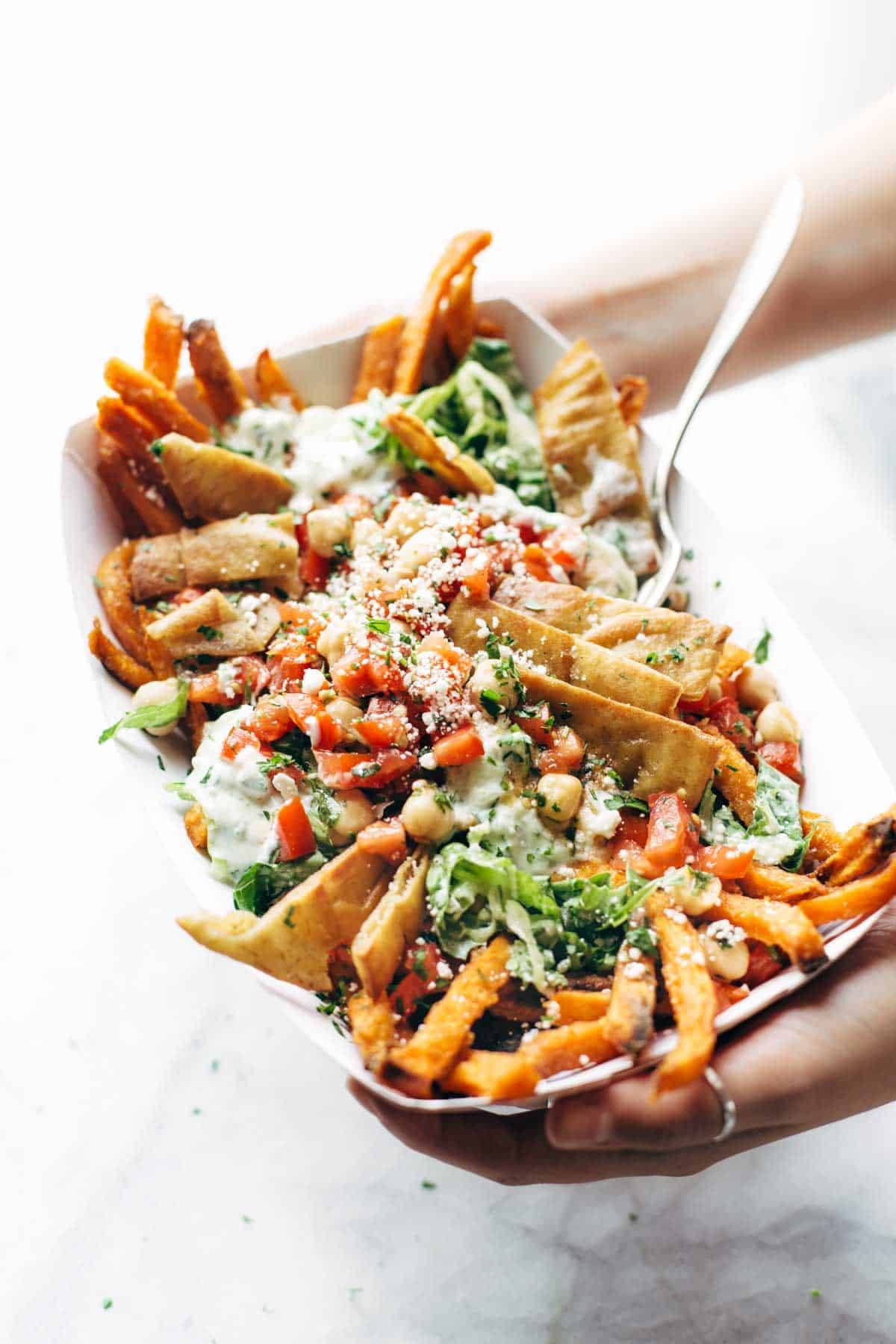This image showcases a vibrant and diverse food dish served in a long, rectangular white bowl, held by two Caucasian hands, one visible near the top in the upper right and the other in the lower right, partially cut off at the wrist. The focal point of the photo is the colorful, appetizing contents of the bowl. It features sweet potato fries, pieces of chicken, sliced tomatoes, and chickpeas, all sprinkled with grated Parmesan or feta cheese. There are also some pita chips, possibly mixed with romaine lettuce, and a hint of a thick white dressing, which could be ranch or sour cream. A fork is placed within the dish, signifying its readiness to be enjoyed. The background is predominantly white, suggesting an indoor setting, with a small patch of gray stone pattern in the lower right corner, adding a subtle contrast to the composition.